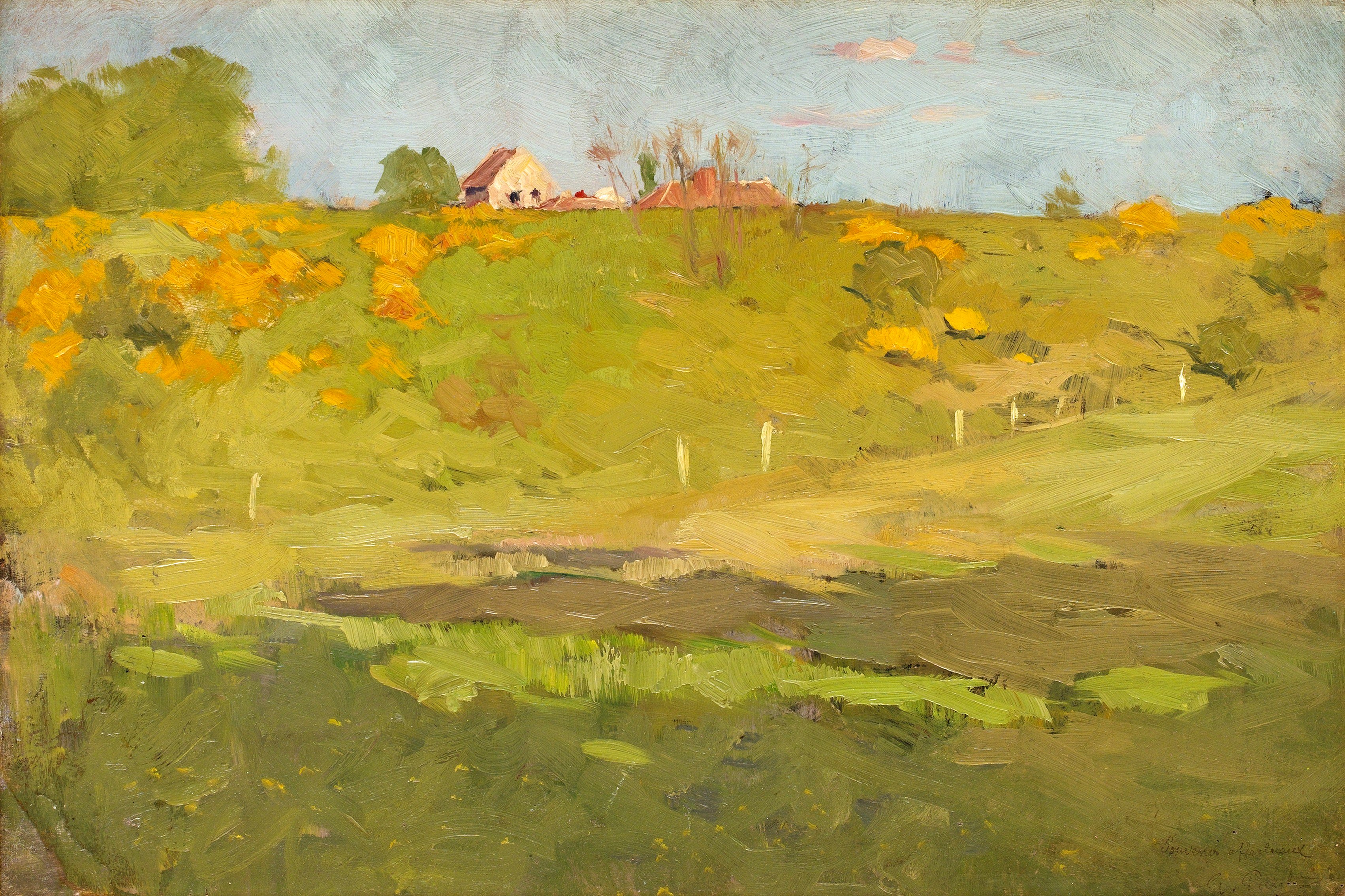This painting depicts a serene rural landscape in a style reminiscent of Impressionism, characterized by broad, explicit brush strokes. The scene captures a vast green field interspersed with patches of yellow and orange, suggesting the presence of flowers or the changing seasons. Towards the field's far end, a series of white fence posts form a boundary. In the middle distance, atop a gently sloping hillside, stands a small house with a cream-colored facade and a brown slanted roof featuring two windows. The hill is dotted with green bushes and a few dormant trees, particularly prominent on the right. The sky occupies the top fourth of the painting, painted in a captivating blue with a few white clouds and extending seamlessly to the field below. The overall composition is in landscape orientation, and the array of colors and textures brings out the vibrancy and tranquility of the countryside scene.